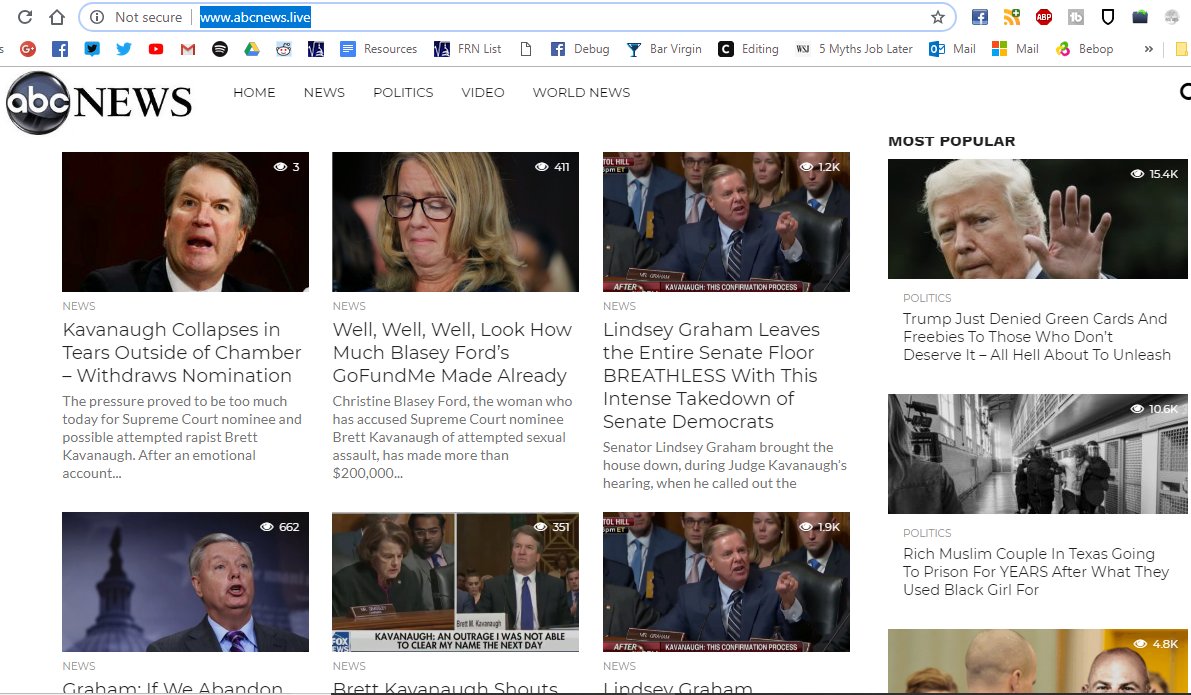This image, sourced from the abcnews.com website, captures a search query at the top, either "abc" or "www.abcnews.live." The screen features a navigation bar with various clickable sections. Prominent images accompany each article down the page.

At the top, under the 'News' section, there's a striking image of an angry man yelling. The headline reads, "Kavanaugh collapses in tears outside of chamber, withdraws nomination." Adjacent to this, another image showcases a woman crying, with the caption, "Well, well, well, look how much Blasey Ford's GoFundMe made already."

Further down, a picture shows a man pointing amidst a group of formally dressed individuals. This image's headline states, "Lindsey Graham leaves the entire Senate floor breathless with this intense takedown of Senate Democrats."

As you continue scrolling, other headlines are partially visible. One reads, "Graham if we abandon," another says, "Brett Kavanaugh shouts," and yet another starts with "Lindsey Graham" but cuts off.

Finally, a popular article discusses a recent statement by Trump: "Trump just denied green cards and freebies to those who don't deserve it. All hell is about to unleash." The page continues further with additional content.